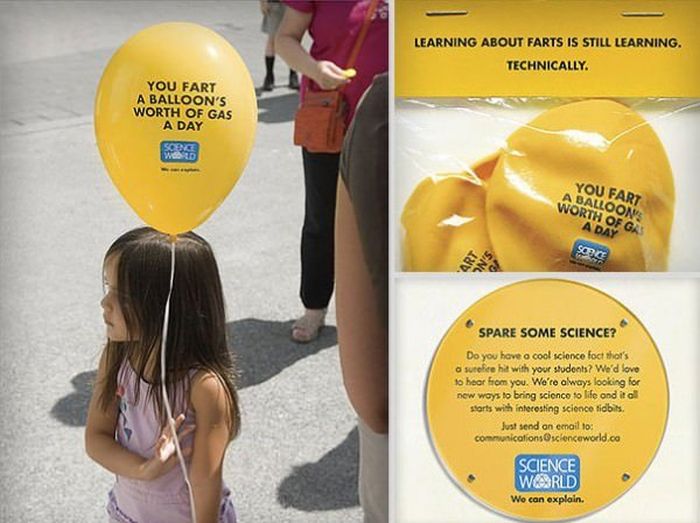The image is composed of three distinct photos arranged in a grid: one large image on the left and two smaller images stacked on the right. The main image on the left features a young girl with straight hair, wearing a pink tank top and gray shorts, holding a yellow balloon. The balloon has the text, "You fart a balloon's worth of gas a day," written in capital letters. She stands on gray asphalt with shadows cast around her, indicating other people nearby. One person in the background wears sandals, black pants, and a reddish burgundy top and appears to be holding something. Another individual is visible in gray shorts, black socks, and black shoes, with an arm extended from someone in an olive green shirt also visible.

In the upper right corner of the image, there's a close-up of deflated yellow balloons inside clear plastic packaging. The packaging has the same text as the balloon held by the girl and is secured with two staples. The text on the packaging reads, "Learning about farts is still learning, technically," over a yellow background.

In the lower right corner, a circular plaque features an appeal for science facts: "Spare some science? Do you have a cool science fact that's a surefire hit with your students? We'd love to hear from you. We're always looking for new ways to bring science to life. Just send an email to communications@scienceworld.co." Beneath this text is the Science World logo in white letters over a blue background, accompanied by the tagline, "We Can Explain." The predominant colors in the image are tan, gray, yellow, blue, pink, red, white, and black, suggesting a vibrant, educational theme aimed at engaging students.